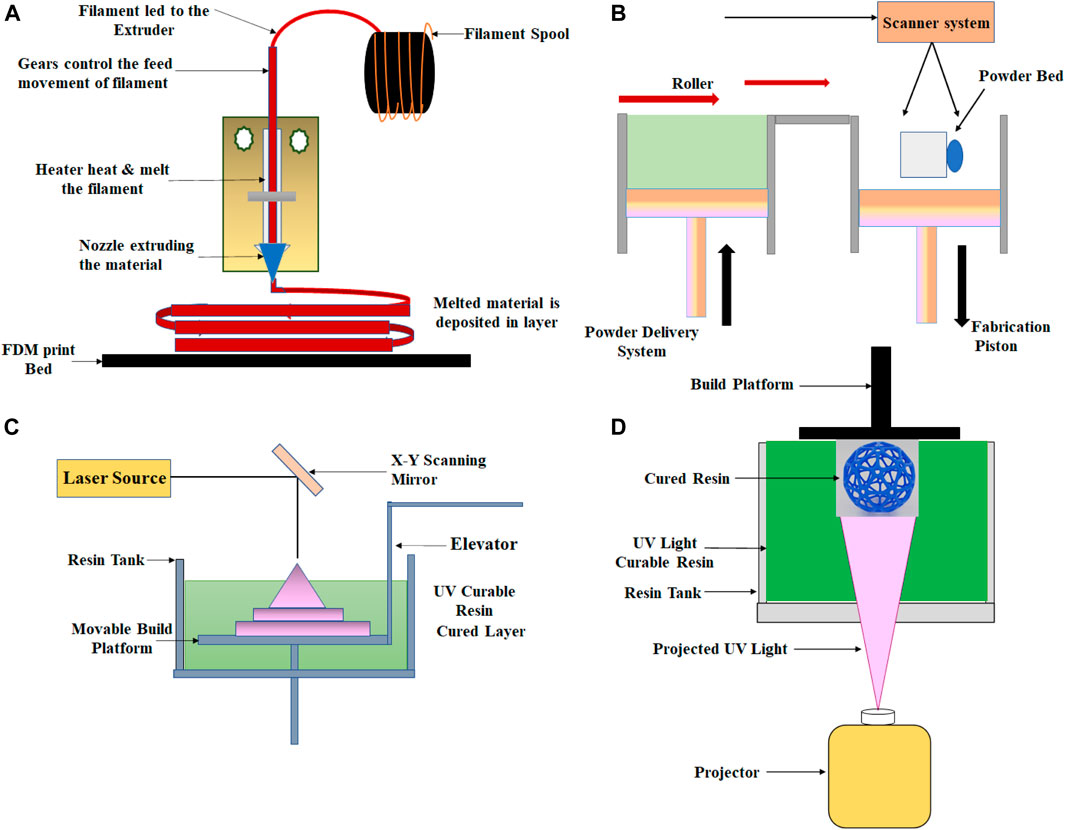The image is a detailed diagram explaining the workings of four different systems, each labeled A, B, C, and D, against a solid white background. 

In section A, a black cylinder or ball is depicted with a spiraling red wire leading into a thicker red line inside a square. This connects to a blue triangle, followed by another spiraling red line. The text explains the parts: a filament spool, filament lead to the extruder, gears controlling the filament's feed movement, a heater melting the filament, and a nozzle extruding the material. It refers to an FDM print bed where the melted material is deposited in layers.

Section B, located on the right, shows components of a scanner system. It includes labeled parts such as a roller and a powder bed, with arrows indicating the flow or movement between these elements.

In section C, the diagram features a square container filled with a green liquid, highlighted by various shapes in purple. Text labels include a laser source, elevator, and UV-curable material, indicating processes likely related to a liquid-based system.

Section D describes another system with a mix of colors and shapes. The parts include a green square, a purple triangle, and text pointing to a build platform, cured resin, a UV light source, a resin tank, and a projector for projected UV light.

Overall, while each section describes different systems, common terms such as UV light, cured resin, and movement controls suggest that all systems might be related to 3D printing or material extrusion technologies.